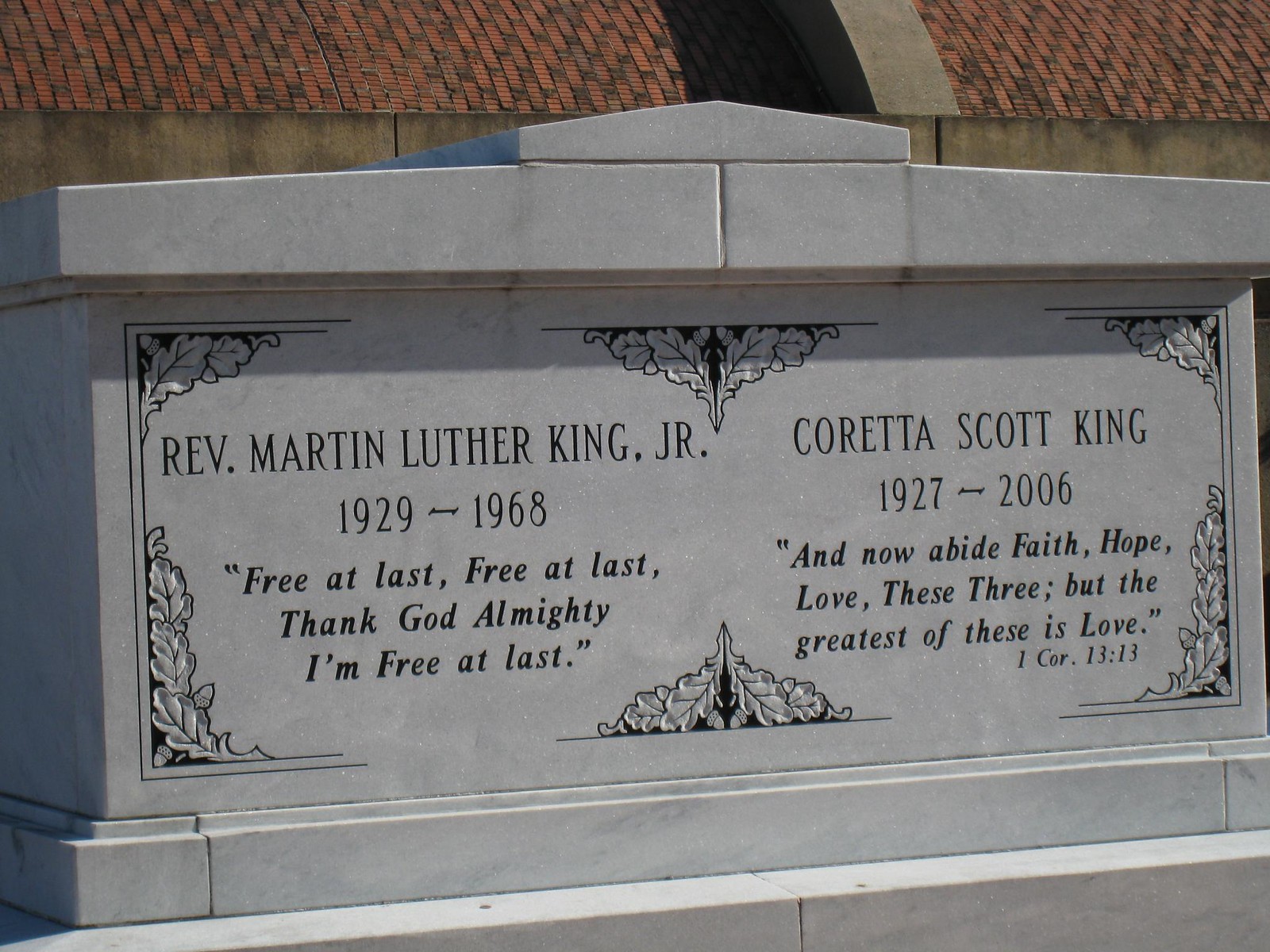The image displays the large, gray tombstone of Reverend Martin Luther King Jr. and Coretta Scott King. Situated side by side, the left side of the tombstone bears the inscription: "Reverend Martin Luther King Jr., 1929 to 1968," with the famous quote beneath it: "Free at last, free at last, thank God Almighty, I'm free at last." On the right side, it reads: "Coretta Scott King, 1927 to 2006," accompanied by the Bible verse: "And now abide faith, hope, love, these three; but the greatest of these is love. 1 Corinthians 13:13." The tombstone features detailed carvings on its corners around their names. There is some sentiment that the image might appear somewhat animated or digitally created, giving it a slightly surreal look, although the inscriptions remain clear and historically significant.